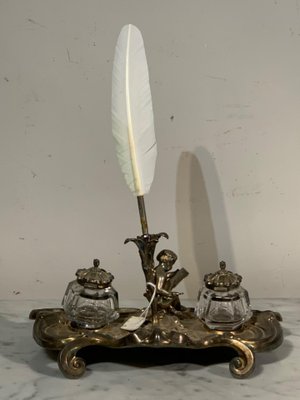The image depicts a well-preserved antique desk inkwell set, attributed to Charles X from the 1840s, made of silver-plated bronze. The central piece is a slightly weathered, ornate bronze statue featuring a boy reading a book. This central figure functions as the holder for a white feather quill pen, which is oval in shape and prominently placed in the middle. The base, resembling a platter with intricate, decorative feet, supports two clear glass ink vessels on either side of the statue, each topped with elaborate metal lids. The set is positioned on a dark gray marble table with a stark white wall in the background, which bears some marks and shadows, including the distinct shadow of the quill pen.